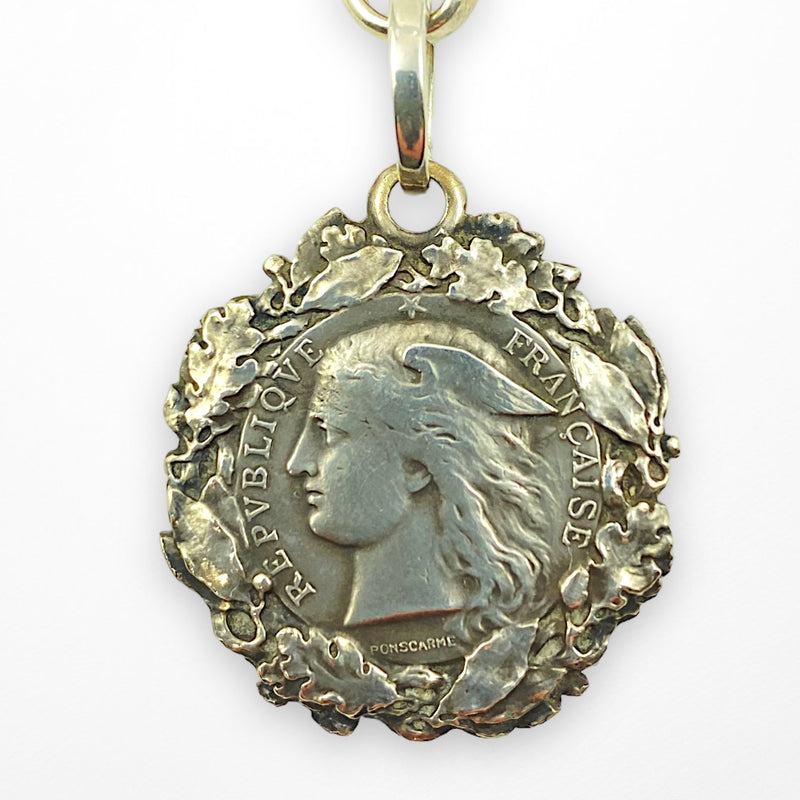This close-up image captures a detailed view of a silver amulet or pendant designed to be worn on a chain, evident by a hook at the top. The background of the image is a light green surface, providing a gentle contrast to the silver, slightly greenish-gray hue of the pendant. The pendant itself is mostly round with an intricately patterned border resembling leaves. 

At the center of the pendant is a circular ring that encases the side profile of a figure with long, straight hair and a notable crown or wings above their head. The figure has large, open eyes, a prominent nose, a small mouth, a pointy chin, and a rounded jaw; their ear is partially visible, and the face appears clean-shaven. The neckline of the figure is also visible.

Inscribed along the periphery within the circular band are the words "REP V V L I Q V E Francis" on the right side, and "PONS CARME" at the bottom, suggesting French or Latin origin. A small star is positioned at the top center of the circular ring, further adding to the intricacy of the design.